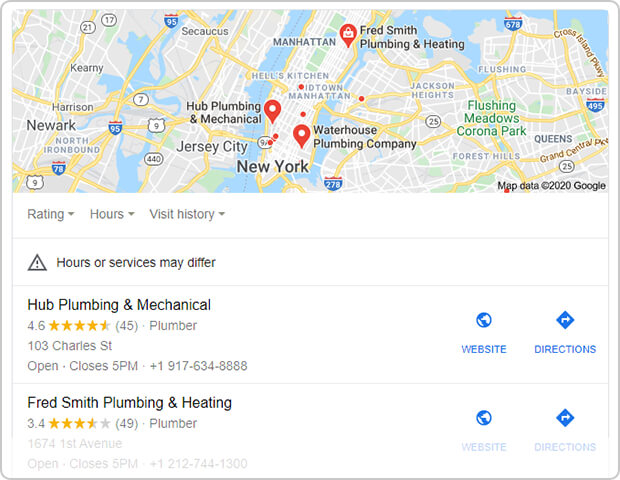A detailed map showcases the area spanning Harrison and the Ironbound neighborhood in Newark to Manhattan, highlighting key landmarks and locations. The map includes a copyright notice from Google dated 2020. 

Highlighted businesses on the map:
1. **Waterhouse Plumbing Company**: Located at 103 Charles Street, this plumbing establishment operates from 9 AM to 5 PM and can be reached at +1 (917) 64-8888. It boasts an impressive rating of 4.6 stars from 45 reviews. Their website provides additional details and directions.
2. **Advancement Plumbing & Heating**: This service operates with a slightly lower rating of 3.4 stars from 49 reviews and is available until 5 PM. They can be contacted at +1 (212) 744-1300 for further information.

The map also references well-known locales such as Flushing, Flushing Meadows, and Kern Park. Freeways and blue water bodies are depicted but not clearly identified. Additional annotations mention variables such as visiting hours, rating, and plumber services with their respective scores and review counts.

Overall, the map offers a wealth of information, including operational hours, contact details, customer ratings, and locations of important neighborhood plumbing services.